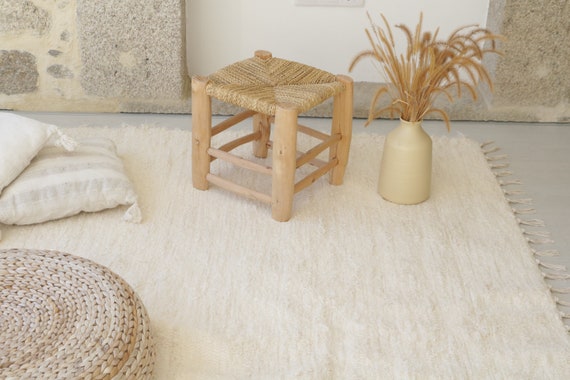The photo captures a serene, minimalist interior, likely within a house, featuring a harmonious blend of light, neutral tones. Centered on a grayish floor is a soft, cream-colored rug, upon which a few carefully selected decor pieces are thoughtfully arranged. A small wooden stool with a woven seat sits next to a beige vase filled with light-colored bamboo stalks, adding a touch of rustic charm. The arrangement includes a round, hand-woven pillow in earthy tones and two square, white pillows adorned with tassels at each corner; one pillow is solid white, while the other features subtle stripes. The backdrop is a textured stone wall, composed of various shades of brown and tan rocks, completing the natural, cozy ambiance. The scene evokes the aesthetic of a modern, bohemian living space, characterized by its clean lines and soothing color palette.